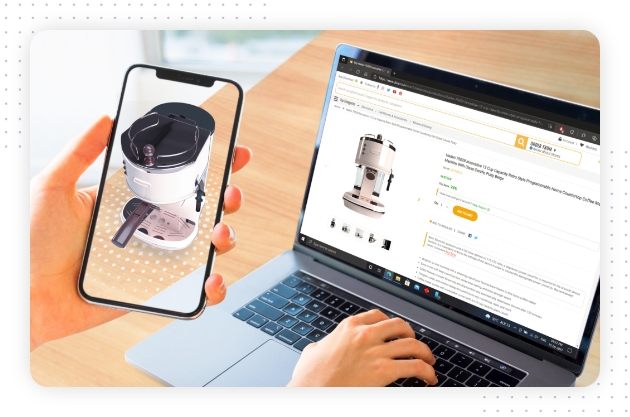The image depicts a person engaged in an online search on a silver-gray laptop with a black keyboard, likely running a Windows operating system. Positioned on a light beige wooden desk, the laptop screen displays a shopping website, possibly Amazon, showing an espresso machine. The person is actively typing with one hand on the keyboard while holding a smartphone in their left hand. On the smartphone, an image of a different, yet similar, espresso machine, with a white body and black lid, is visible. This suggests the person is comparing the two devices. The background features a faint glimpse of a stainless steel appliance, possibly an oven.